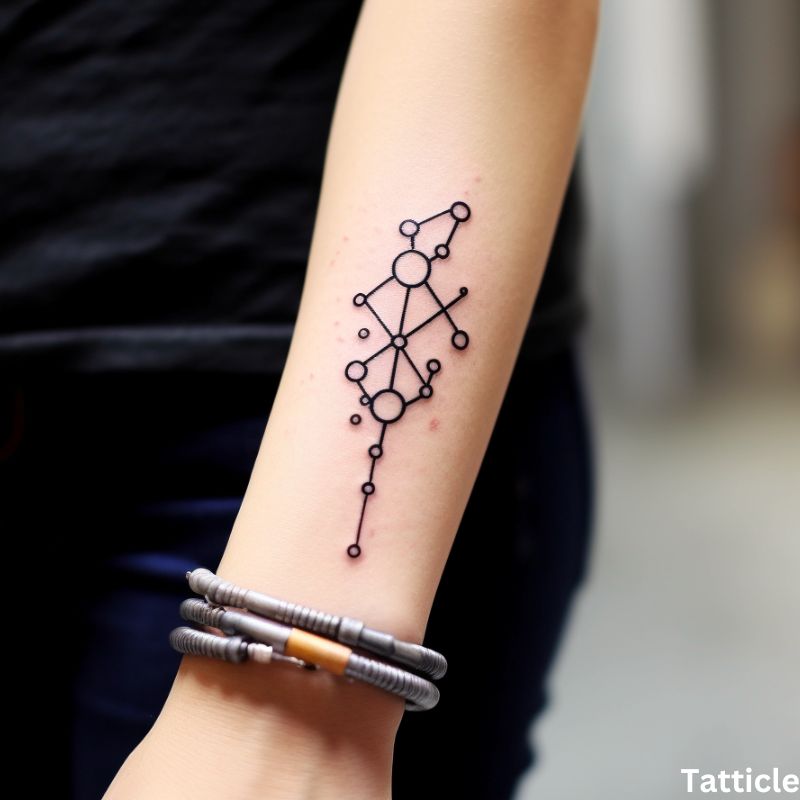The photograph captures the left arm of a young woman adorned with a tattoo and a bracelet. The tattoo, located on the underside of her arm, features a pattern of interconnected circles and lines, possibly representing circuits or an abstract design. The tattoo's skin appears slightly raised, suggesting it might be fresh. The arm itself is pale and extends from the bottom middle, left a bit, up to the top middle of the image. The word "Tactical" is inscribed on the lower right part of the arm. The woman's bracelet resembles a coaxial wire with a visible connector near her wrist.

She is wearing a black shirt and dark blue jeans. The background is blurry, with more noticeable blur on the right side of the image. The colors in the picture include beige, black, a yellowish copper shade, gray, and blue. Light appears to be coming from the top, highlighting the bracelet and the tattoo. The setting focuses on showcasing the tattoo on her left arm amid the out-of-focus backdrop.